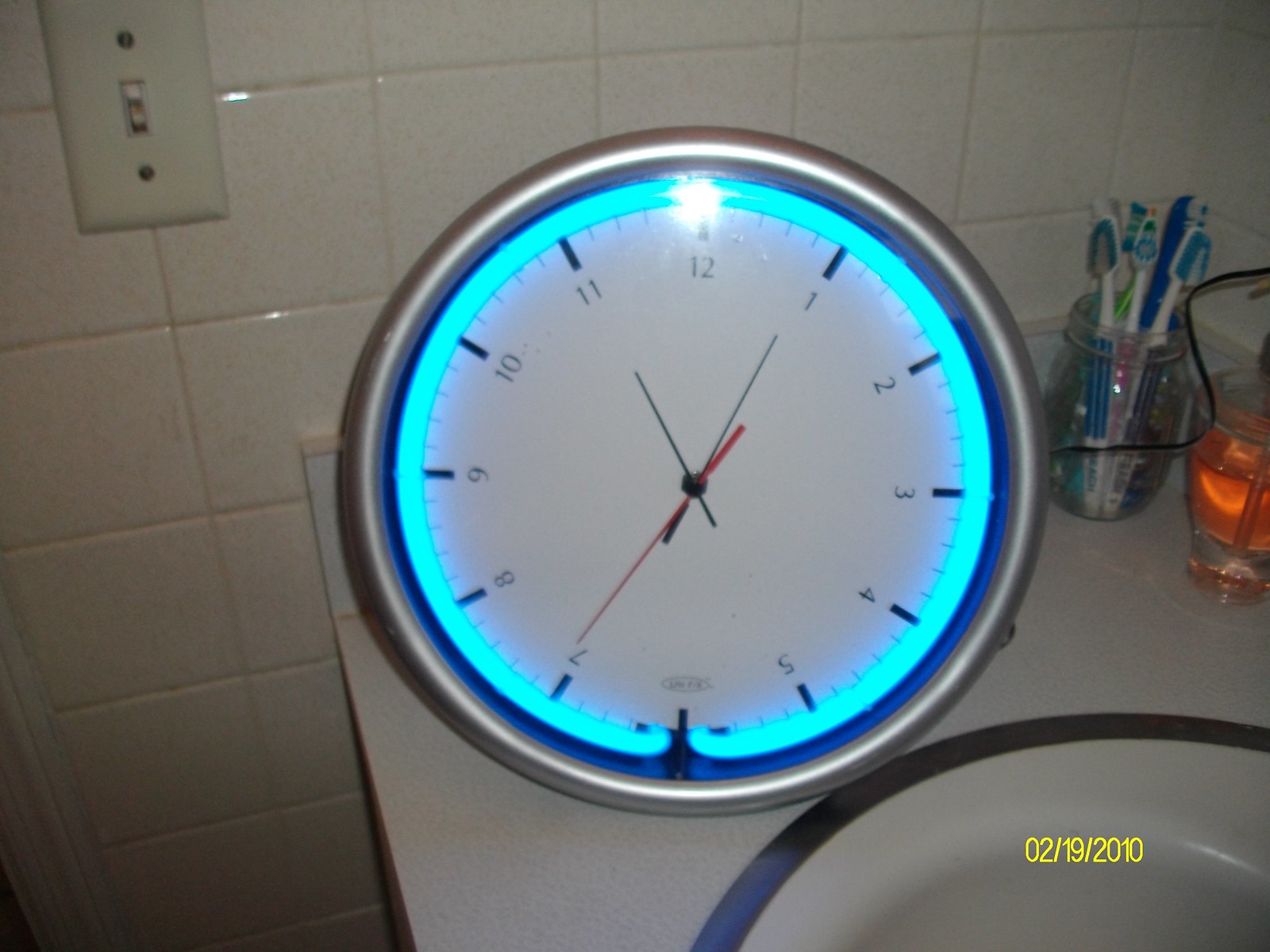This color photograph captures a detailed scene in a bathroom, centered around a round, silver-framed wall clock resting on a white sink. The clock, which displays the time at 11:04, features a white face with black hour and minute hands, a red second hand, and blue numbers. The standout detail is the neon blue ring of light that backlights the clock’s edge, giving it a striking appearance.

The clock leans against a wall made up of white square tiles with white grout, and there's a white light switch on the left side of the wall. On the right side of the sink, there's a clear glass jar filled with variously colored toothbrushes—pink, blue, white, green, and turquoise—suggesting a family bathroom. Additionally, an orange object that resembles a candle sits beside the jar.

Noteworthy is a navy stripe that encircles the outer edge of the white sink, adding a touch of color contrast. The image also includes a dated timestamp in the bottom corner, marked "02/19/2010," adding a historical context to the photograph.